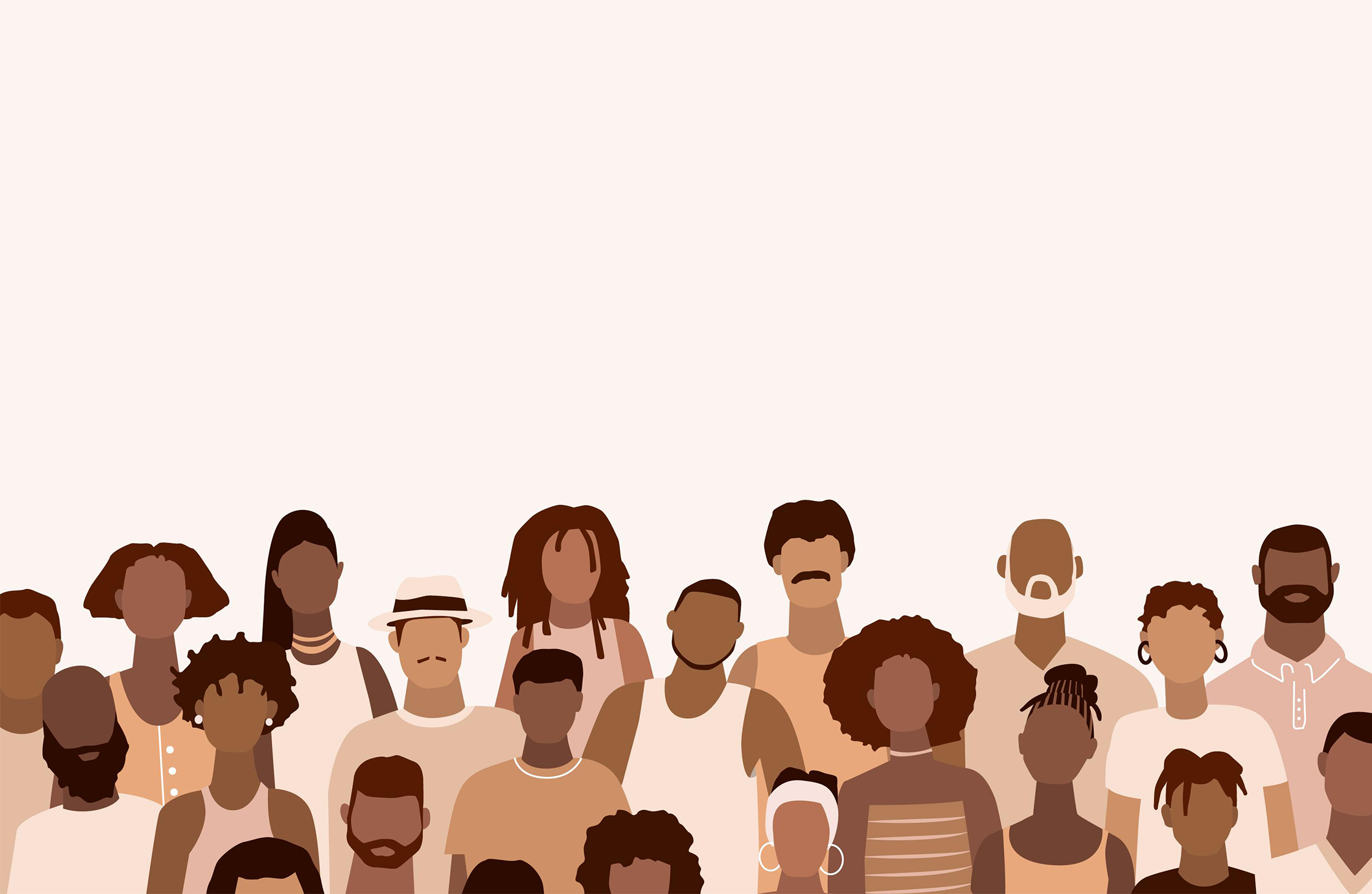This is a detailed clip art illustration depicting 22 people of varying genders and skin tones, from light to dark brown. All individuals are shown from the neck or chest up against a solid light salmon background. None of the figures have facial features, such as eyes, noses, or mouths; however, some males display mustaches or beards. The group showcases a range of hairstyles including long locks, short cuts, braids, afros, and dreads. Attire includes casual clothing with combinations of white, light peach, cream, and pinkish-colored tops, some adorned with collars, stripes, or jewelry. Notable details include a woman with short brown hair, a woman in a white sleeveless top with a necklace, a man with a hat and mustache, and several other figures with distinctive hairstyles. The illustration also includes elements like hats and earrings that add to the diversity and individuality of each character.